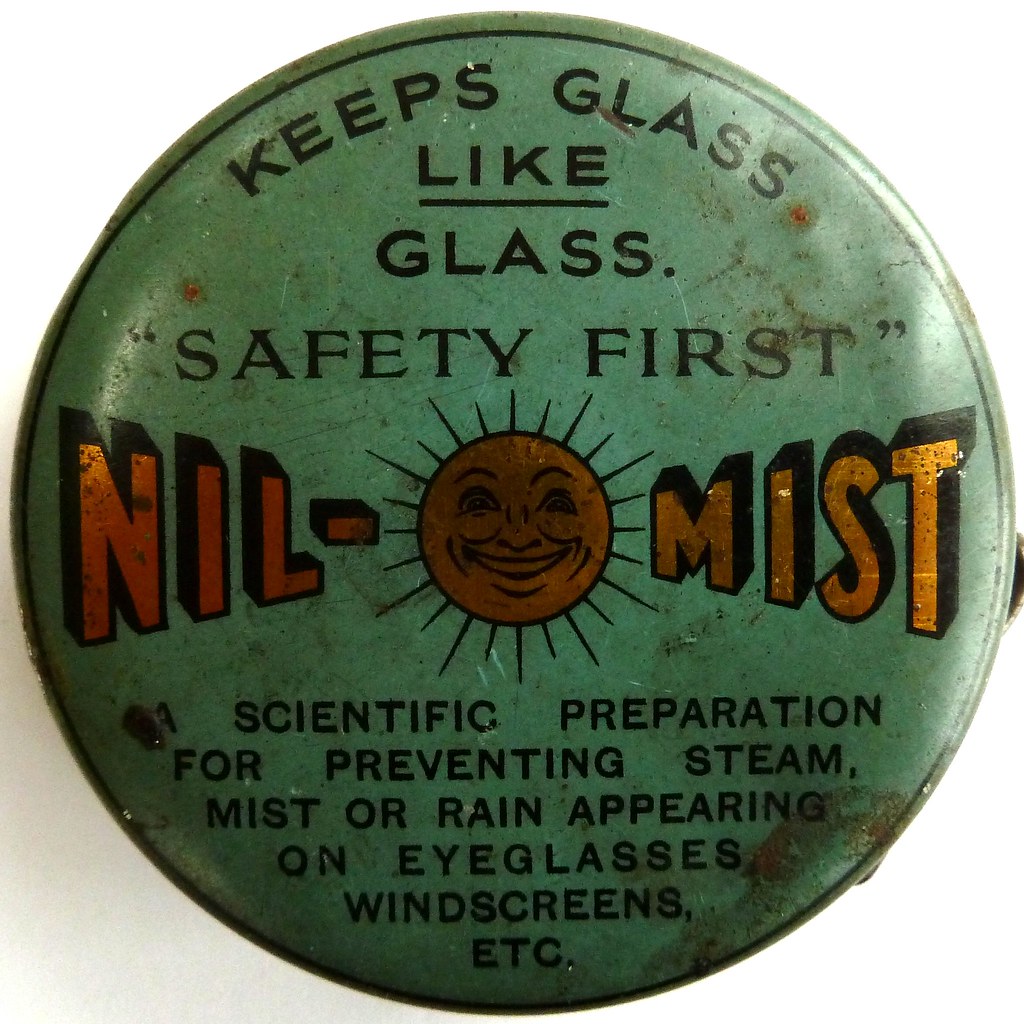This image features the top of an old, circular metal tin that exhibits significant wear and traces of rust, indicating its antique nature. The tin is primarily green, though aged, and adorned with black text. The topmost text reads, "keeps glass like glass, safety first." At the center of the tin is a depiction of a smiling sun, rendered in a coppery gold color and outlined in black. Flanking the sun, bold black-bordered letters spell out "NIL" on one side and "MIST" on the other, arranged to add visual weight and texture. At the bottom, the tin is inscribed with detailed black text that reads, "a scientific preparation for preventing steam, mist, or rain appearing on eyeglasses, windscreens, etc."